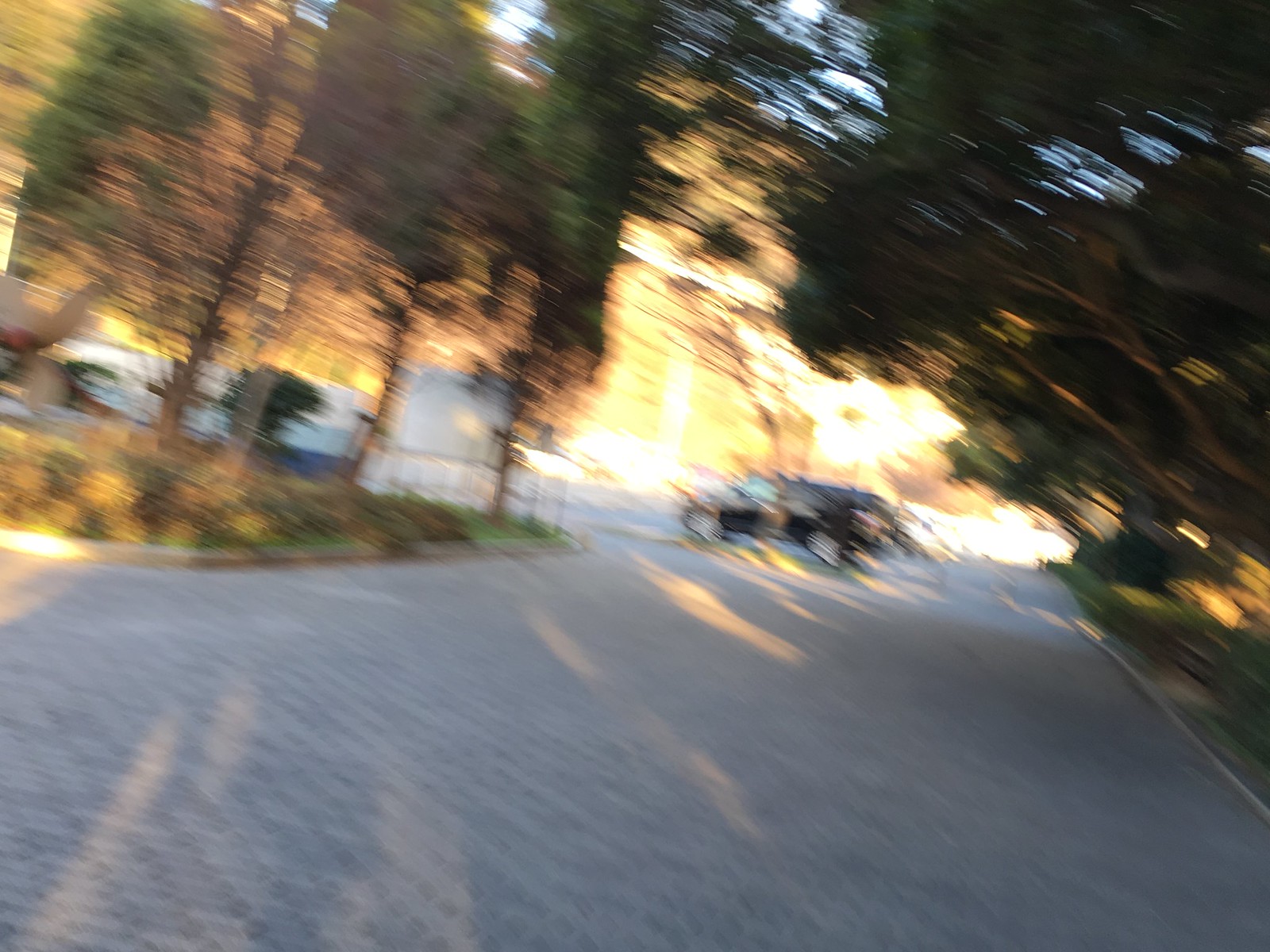The image depicts a parking lot bordered by a stone pathway that leads to a cement area where cars are parked. The scene is set in early fall, as evidenced by the trees that are beginning to turn brown while retaining much of their green foliage. The golden light of the late afternoon sun filters through the trees, casting a warm glow and causing the leaves to appear yellowish. A black van can be seen prominently parked among the vehicles. The overall setting suggests a peaceful time of day, with the sun starting its descent towards the horizon but still providing ample daylight.